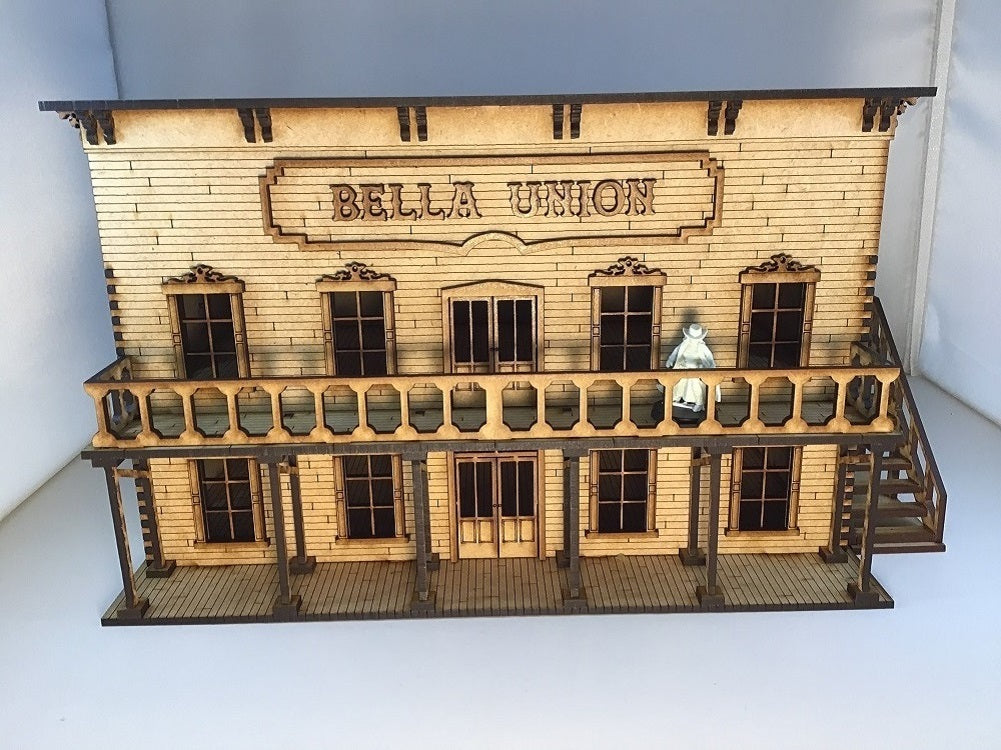This detailed image captures a meticulously crafted miniature model of a 19th-century Western-style building, reminiscent of those seen in old west towns on television. The building, named Bella Union as indicated by the carved wooden sign atop its false brick front, showcases a striking blend of light yellow brick and various shades of brown woodwork. It is a two-story structure with the second floor featuring a comprehensive balcony that stretches across its front, supported by a wooden covered walkway serving as a roof for the first story.

The building’s facade is adorned with a balance of windows and doors: the first floor exhibits a double door entrance flanked by two large windows on either side, while the second floor mirrors this arrangement with a row of five windows and a balcony that runs its entire length. On this balcony, a white carved figure wearing a hat adds a touch of charm and character.

An external staircase extends from the right side of the building, providing access to the second floor, which seems to have another entry point. The intricacy of this model is underscored by the detailed textures of the wood and brick, making it a captivating representation of historical architecture.